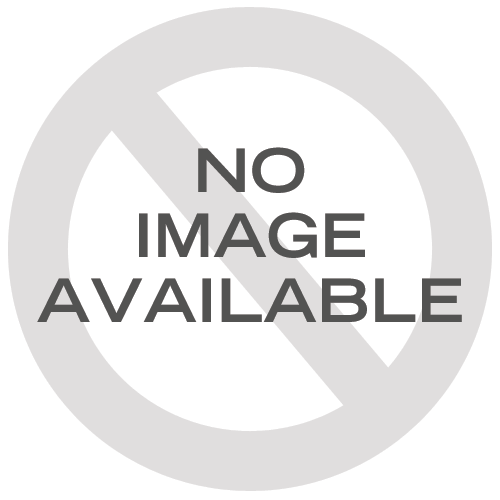The image depicts a standard placeholder graphic commonly used to indicate that no image is currently available. It features a large, solid gray circle outlined prominently in a slightly darker shade of gray. Cutting diagonally across this circle from the top left to the bottom right is a bold gray line. Overlaid in the center of the image, and also centered within the circle, is the phrase "NO IMAGE AVAILABLE" written in a dark gray, uppercase, bold font. The text is presented in three lines: "NO" on the first, "IMAGE" on the second, and "AVAILABLE" on the third, all centrally aligned. The overall design is minimalist, utilizing varying shades of gray to convey the placeholder message clearly and effectively.